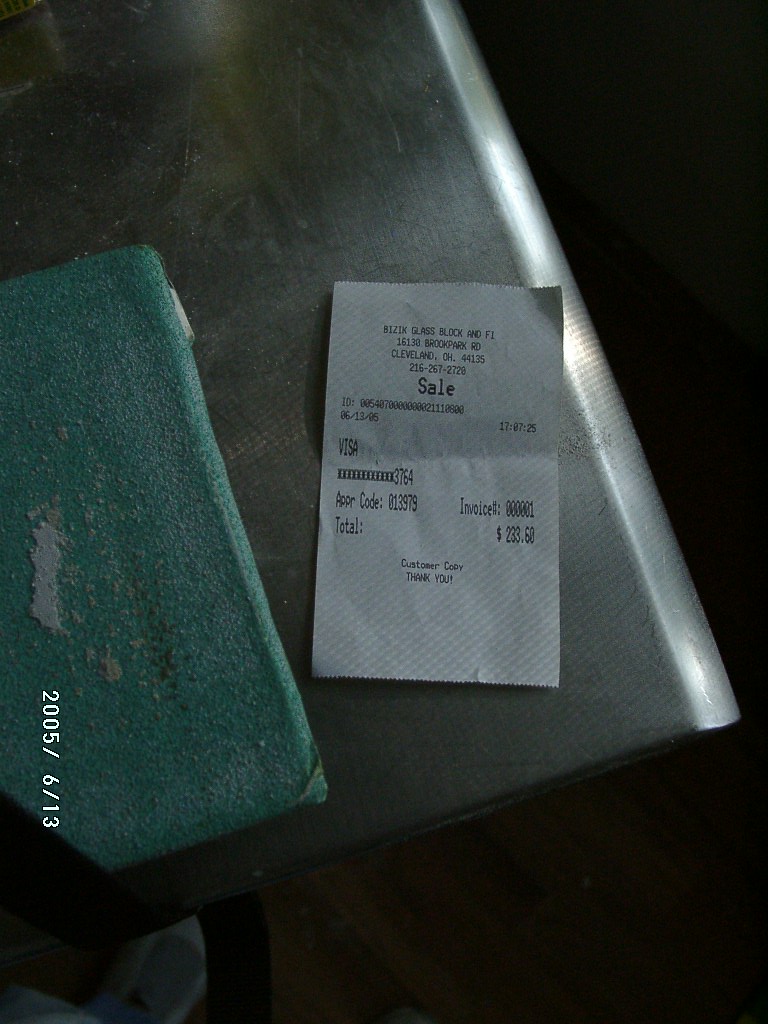This detailed image captures a scene with a stainless steel table, identifiable by the visible leg underneath. The dark brown wooden floor contrasts sharply with the metallic surface. Atop the table lies a small sales receipt, indicating a total purchase amount of $223.50. The receipt features the purchase information at the top and the word "SALE" prominently displayed in bold black letters in the middle. Next to the receipt is a large teal-colored cleaning sponge, smeared with a gray abrasive cleaner. The picture was taken on June 13, 2005.